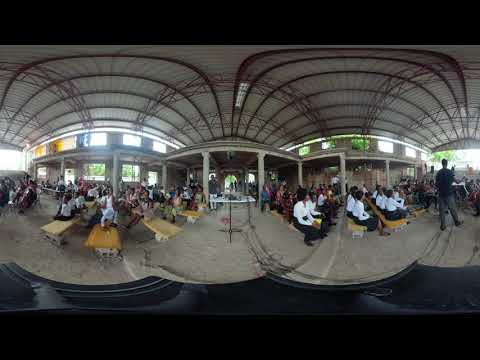The photograph captures the interior of what appears to be a transportation hub, food court, or an educational setting that has a fisheye lens effect. The image showcases wooden benches on both the left and the right sides, with numerous people seated on them. Most of these individuals are wearing white shirts paired with either black pants or blue slacks, adhering to a uniform, signaling a possible student or formal setting. A few people are dressed casually. In the center, a person is seen walking. The floor is light gray, and the ceiling is white with metallic supports. Several windows line the walls, allowing ample sunlight to flood the room. The picture appears slightly distorted, possibly due to the fisheye filter or panoramic stitching, with two horizontal black strips at the top and bottom edges. The overall scene suggests a bustling, sunlit space that serves as a hub for activity, likely in a non-Western country such as India or Malaysia.